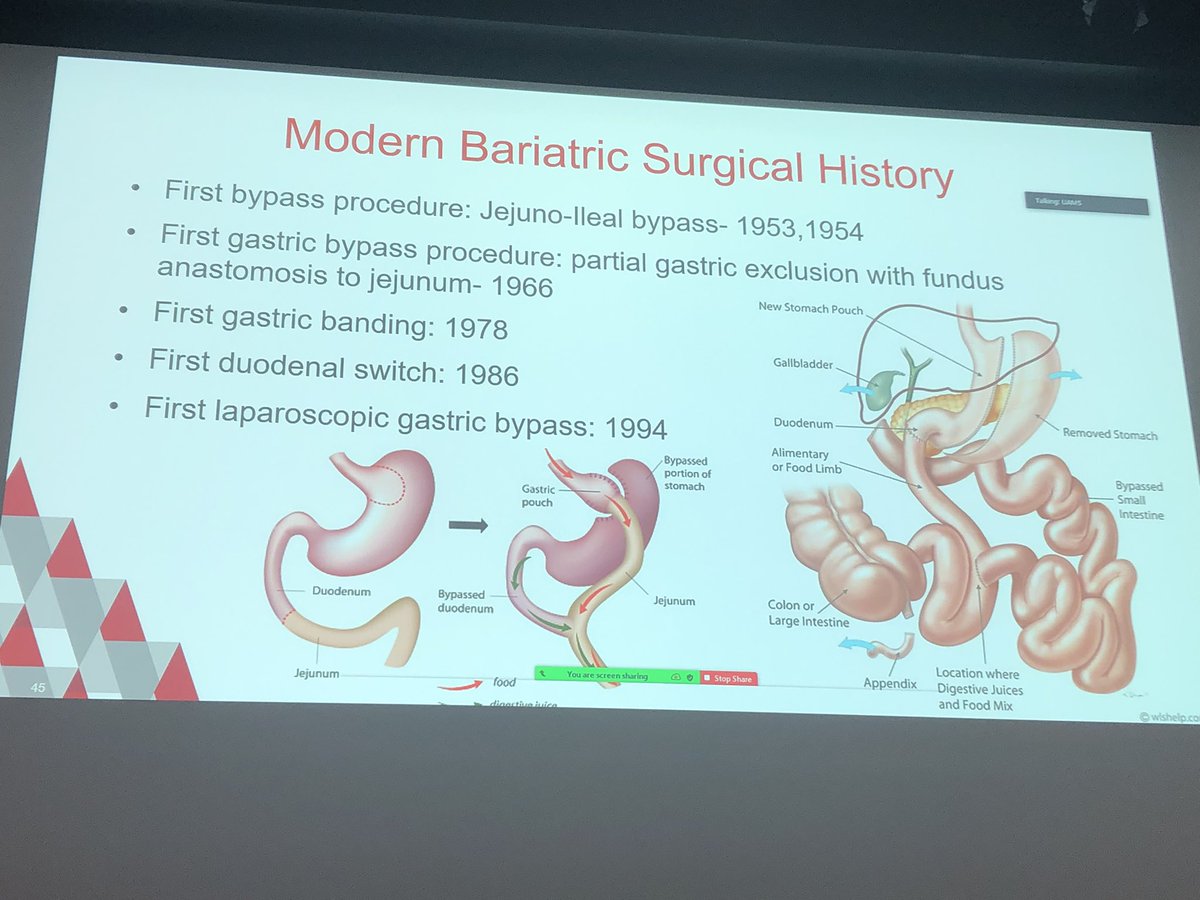The image is a photograph of a computer screen displaying a detailed slide on "Modern Bariatric Surgical History." The slide is framed by a black border and is set against a light sky-blue background with a series of bullet points elaborating on the timeline of bariatric surgical advancements. The title, "Modern Bariatric Surgical History," is prominently displayed in orange at the top. Below the title, key milestones are listed in red text with corresponding years: 

1. First bypass procedure - jejunoileal bypass (1953-1954)
2. First gastric bypass procedure - partial gastric exclusion with fundus anastomosis to jejunum (1966)
3. First gastric banding (1978)
4. First duodenal switch (1986)
5. First laparoscopic gastric bypass (1994)

To the bottom right, the slide features graphic illustrations of the stomach and intestines. These annotated images in peach or pink colors present various stages and techniques of the procedures discussed, such as a jejunoileal bypass, a bypassed duodenum, a gastric pouch, and the modified anatomy post-surgery. The illustrations meticulously label the gallbladder, the new stomach pouch, the removed stomach portion, the duodenum, the alimentary limb, the bypass portion of the small intestine, the mixing point of digestive juices and food, the appendix, and the colon. Furthermore, the bottom left corner of the slide features a design comprising red, gray, and light gray triangles, adding a graphical element to the detailed medical content.